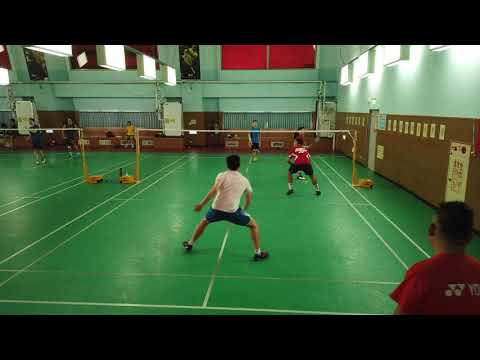In this indoor auditorium, around seven men, possibly in their late teens or early twenties, are engaged in a sport. The vibrant green court, adorned with white lines, is divided down the middle by a yellow and white net, indicating a game similar to volleyball. On the nearest side of the divider, a player in a red shirt and black pants, alongside another in a white shirt and blue pants, can be seen. Further back, another individual in a red shirt is preparing for play. The opposing team on the far side of the net includes players in blue and red shirts, among others. The auditorium's walls feature an earthy brown color on the lower half, transitioning to green above, capped with fluorescent lights hanging from the ceiling. At the back, large windows are covered with red shades. Another court, also green, is visible to the left, with two additional players and another net, creating a dynamic, multi-game environment.